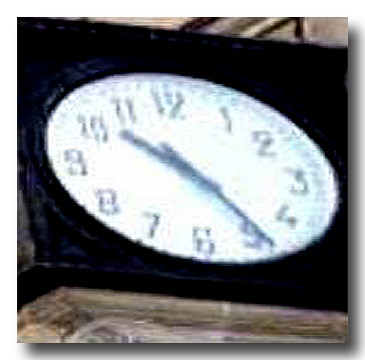This image captures a detailed view of a large clock face, likely mounted on a building or possibly a mantle, although discerning the exact location is challenging. The clock appears to be enclosed in a black frame, with a stark white face that provides a striking contrast. The numerals on the clock are exceptionally large, suggesting that the clock itself is of considerable size. Surrounding the circumference of the clock face, small dots mark each minute. The time displayed is 10:25, with both the hour and minute hands being black. A hint of a stone ledge can be seen at the bottom of the clock, and it is plausible that there is stonework above it as well. The photograph is taken from a lower angle, making the clock seem slightly tilted backwards. This perspective further enhances the grandeur of the clock, reinforcing the impression that it is part of an impressive architectural structure.